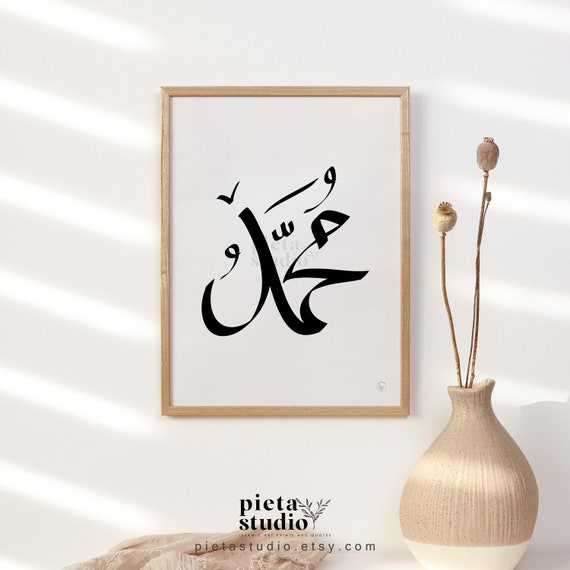The image features a tan and off-white vase with a brown curvy design and three dried flower stems devoid of petals, positioned beside an art piece hanging on a white wall. The art piece, framed in a light wood-colored frame, comprises black script that seems to resemble an Arabic symbol or possibly another language, containing elements that look like the letters V and W. The artwork is paired with multiple lines and a curvy signature. There are bands of light and shading cast against the wall, likely from a nearby window. At the bottom of the artwork, text reads "pietastudio" in all lowercase letters, followed by "pietastudio.etsy.com".